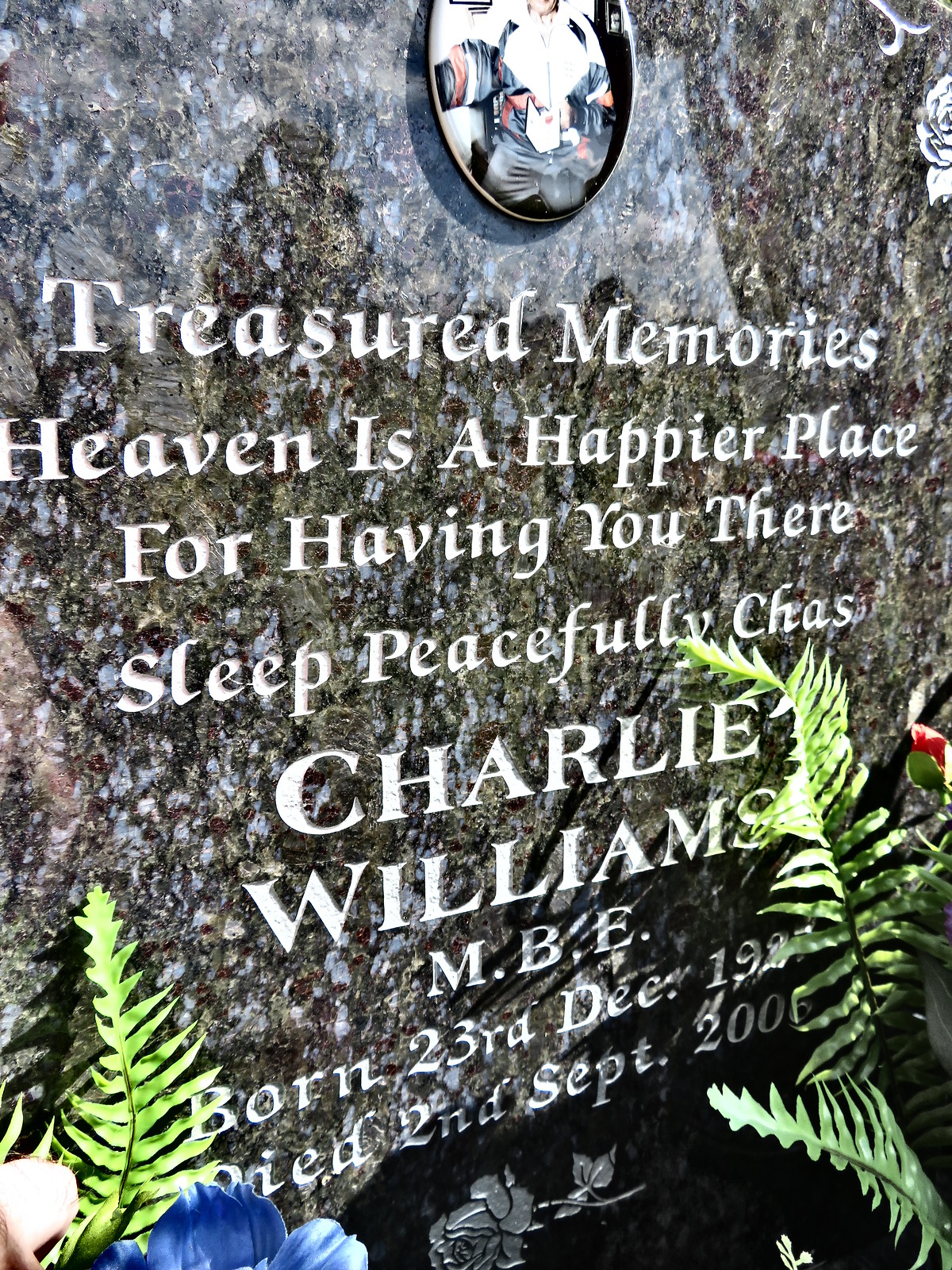The photograph captures a striking marble gravestone of dark brown and gray hues, taken outdoors. Featured prominently at the top is a slightly cropped photo and an oval medallion of the deceased, with the inscription in white lettering beneath it reading, "Treasured memories, heaven is a happier place for having you there. Sleep peacefully, Chaz." The gravestone commemorates Charlie Williams, MBE, with the birth date partially obscured by ferns, only revealing "born 23rd December, 19...," and it clearly states his death on "2nd September 2006." The bottom of the headstone displays an engraved rose. Green ferns frame the headstone, with a blue-petaled flower visible at the lower left-hand corner of the image, adding a touch of color to the somber scene.